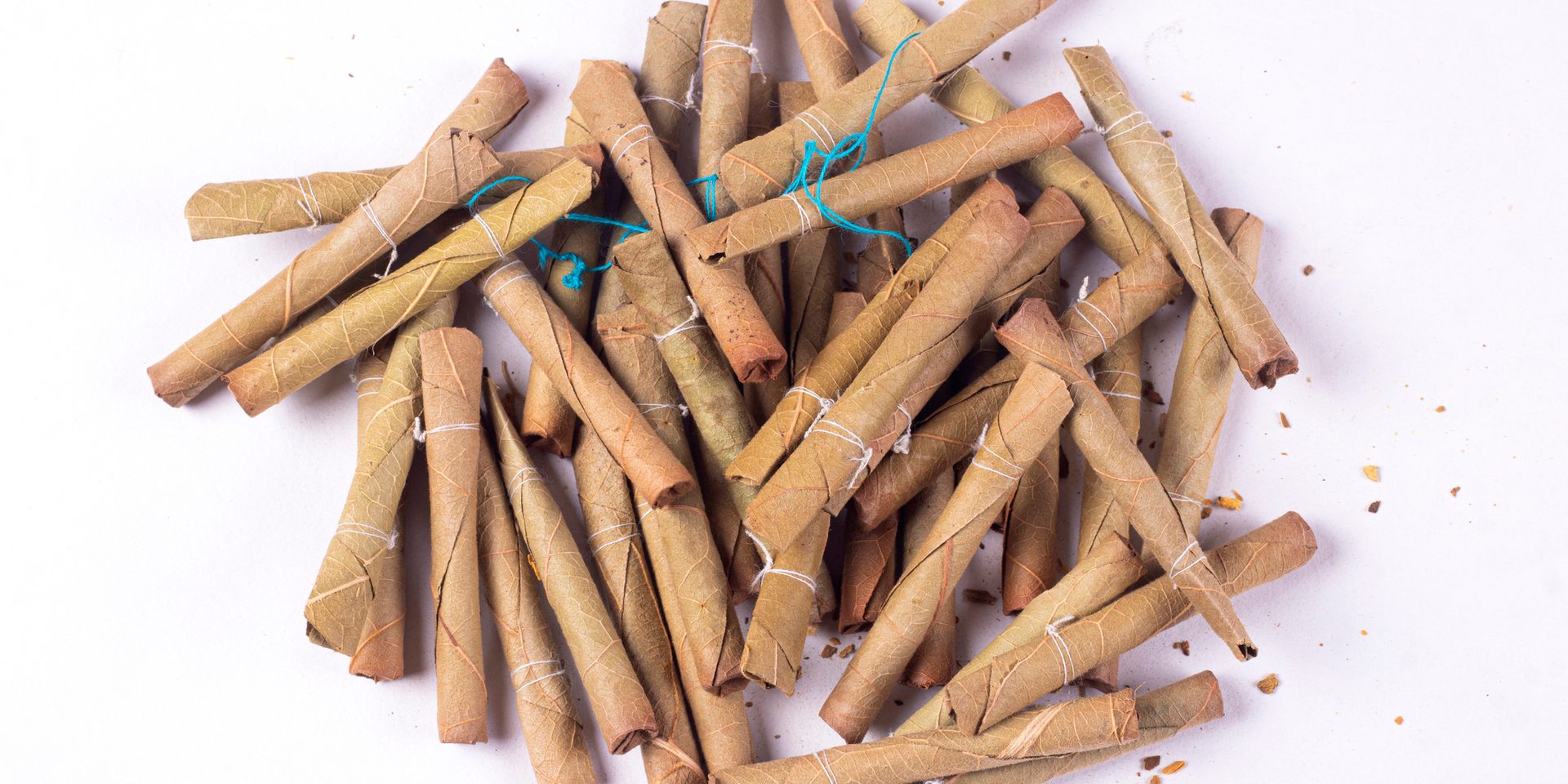This photograph captures a detailed and intriguing view of a pile of rolled-up leaves against a pristine white background. Each leaf is meticulously wrapped into a small, tightly bound roll, somewhat comparable in size to a cigarette. These rolls are secured with thin threads, predominantly white, although a few are tied with blue thread. Scattered beneath the pile are bits of crumbled leaf fragments, adding texture and complexity to the scene. The leaves appear to be tan or brown in color, and despite their careful preparation, there is no distinguishing information available about their origin, purpose, or the person responsible for gathering and rolling them. The image provides a close-up perspective, highlighting the intricate details of the stems and the craftsmanship involved in binding the leaves.